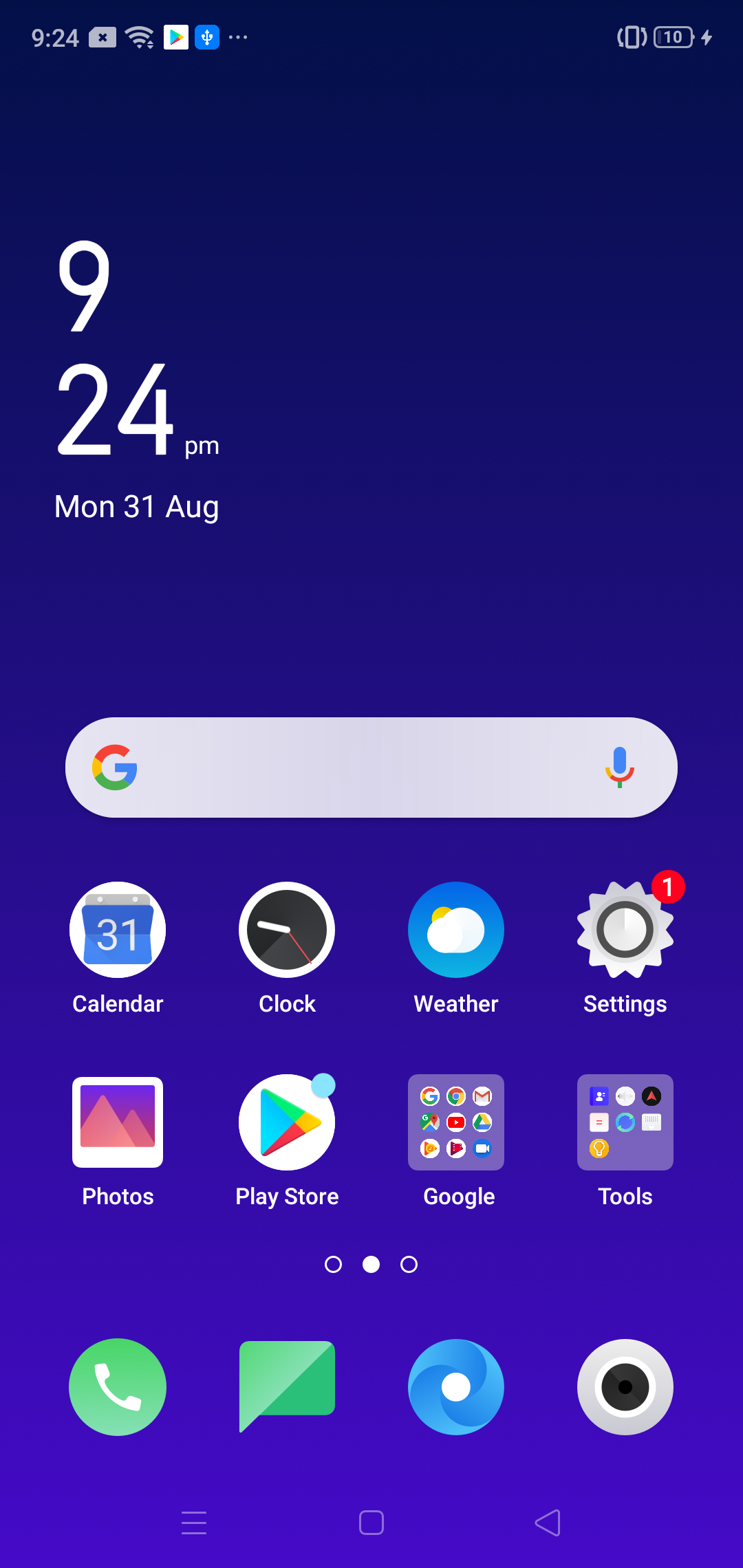The image depicts a smartphone's home screen interface, presented in a vertically long and tall format. In the top left corner, the screen shows the current time, "9:24," next to various status icons including an SD card symbol, a WiFi symbol, a Google Play icon, and a blue Ethernet-like symbol. On the top right, the interface displays a battery icon indicating a 10% charge, with a small lightning bolt symbol signifying it is charging.

Beneath these icons, in white text, the device shows "9:24 PM, Monday, 31st August" against a bluish background that darkens towards the top. Below the time and date, there is a prominent Google search bar.

Further down, a row of app icons is visible, starting from left to right:
- A calendar app icon marked "31."
- A clock app icon featuring a black clock face.
- A weather app icon showing a cloud with a sun peeking from behind.
- A settings app icon represented by a gear with a red notification badge.
- A photos app icon displaying a stylized picture.
- The Play Store icon in the shape of a colorful triangle.

Additionally, two folders are visible:
- A "Google" folder containing multiple icons.
- A "Tools" folder also containing several app icons.

At the bottom of the screen, a dock houses four more app icons:
- A green phone dialer icon.
- A green messaging speech bubble icon.
- A blue swirl icon, potentially representing a browser or an app.
- A camera icon resembling a camera lens.